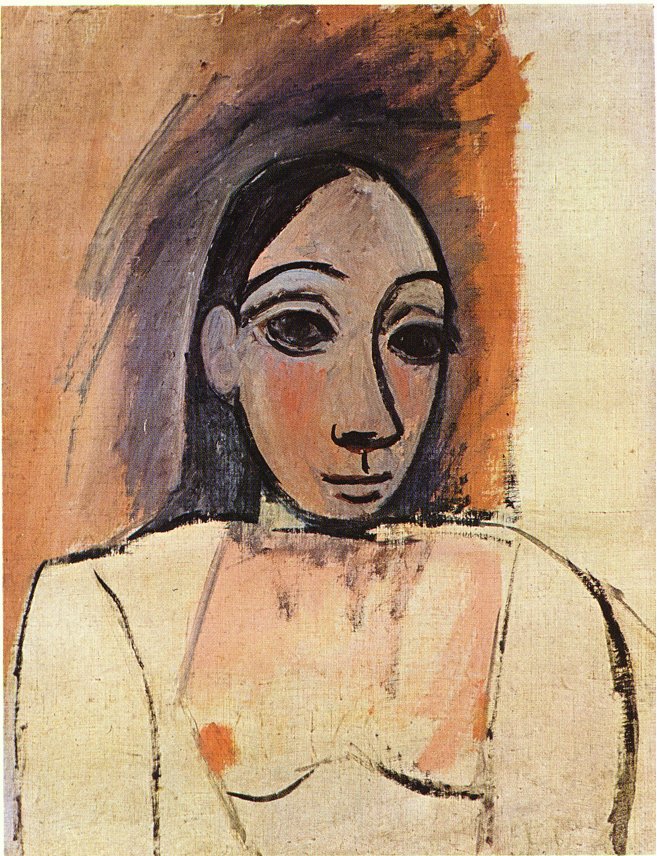The artwork depicts a crude yet captivating sketch of a woman, with her features vividly painted or colored in. The canvas has a rough texture in a tan shade. The background to the right is predominantly white, transitioning into vibrant hues of yellow and orange on the left, accented by sporadic black streaks.

The woman, likely an African American or Indian, has a distinctly oval face outlined in bold black, with pronounced, large black eyes and defined pupils. Her dark skin tone is highlighted by subtle hints of peach on her cheeks and blue above her eyes, resembling eye shadow. She wears a suit-like coat, varying between white and tan shades. Her torso, shown down to just below the chest, reveals lighter skin, and at the very bottom of the frame, there are artistically depicted nipples.

Her hair is long, black, and slick, smoothly brushed back behind her ears. The woman’s facial features include accentuated eyebrows, an angular nose, and a straight-line mouth with a smaller line indicating her lips beneath. The overall image combines abstract elements with a more detailed depiction of her face, creating a striking and textured representation.